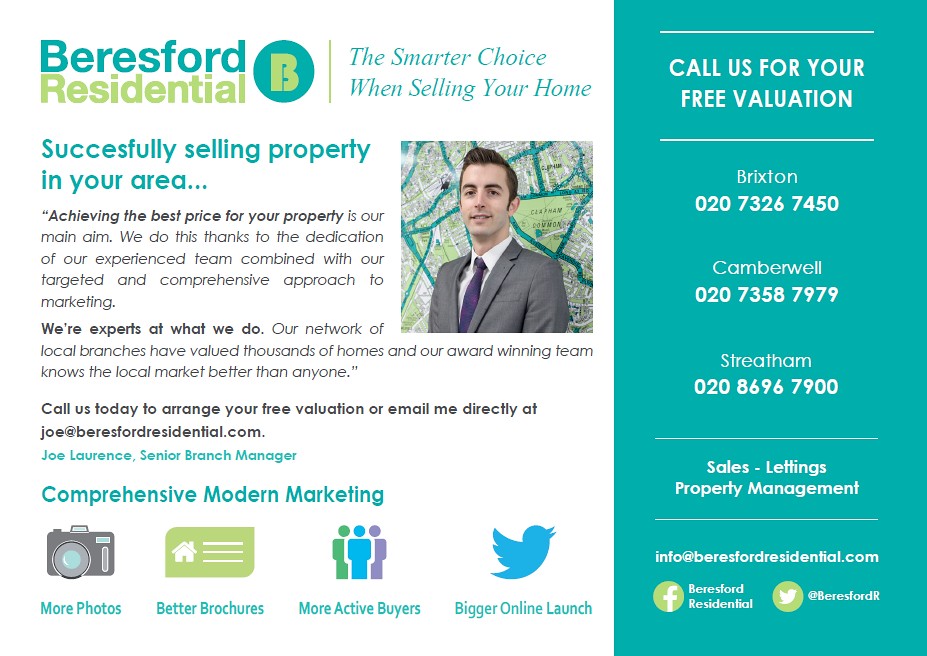The image is a detailed advertisement for Bearfall Residential, a real estate company focusing on sales, lettings, and property management, presented with a comprehensive modern marketing strategy. The central figure in the image is a young man dressed in a gray suit, white shirt, and purple tie, posing against a backdrop resembling a city map filled with streets and parks. The company's name, Bearfall Residential, is prominently displayed on the top left in a blue and green color scheme. Below this, a variety of text highlights their services, emphasizing features like more photos, brighter brochures, more active buyers, and a bigger online launch. Additionally, social media or webpage links and contact information for their branches in Brixton (020 7326 7450), Camberwell (020 7358 7979), and Streatham (020 8696 7900) are accessible through a blue banner on the right side of the image. Various logos and a tagline indicating the smarter choice to sell your home with the offer of a free valuation complete the advertisement.